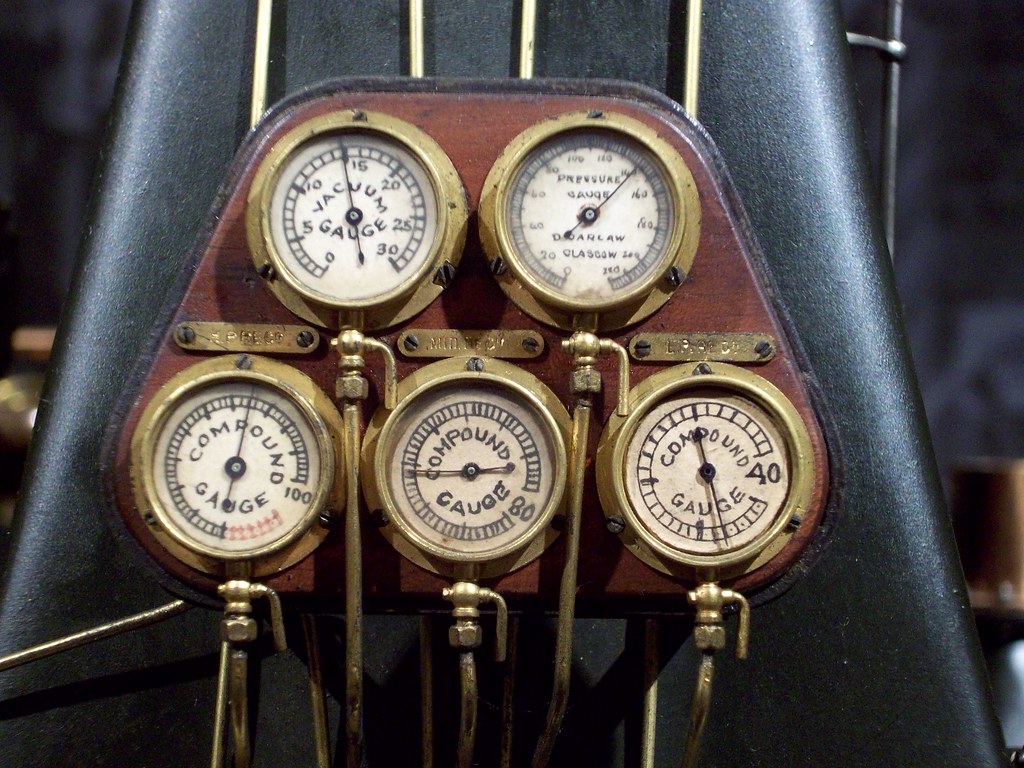This image captures a meticulously detailed view of a vintage industrial instrument panel, likely from a factory or workshop setting. At the heart of the photograph, set against a blurred black triangular backdrop, is a trapezoidal wooden panel mounted on a larger black apparatus. This wooden panel features five brass gauges with white faces, black needles, and black text. The gauges are smartly arranged in two rows—two at the top and three below. 

The leftmost gauge on the top row is labeled "Vacuum Gauge," while the gauge to its right is marked "Pressure Gauge." The bottom row consists of three "Compound Gauge" meters. All gauges are surrounded by gleaming brass edges, and they are connected to a network of brass tubes that descend from them, contributing to the intricate industrial aesthetic.

Additional copper and bronze fixtures can be discerned in the blurred background, enhancing the vintage, mechanical ambience of the scene. The entire assembly is framed by four prominent vertical brass pipes, adding to the complexity and historical charm of the machinery.